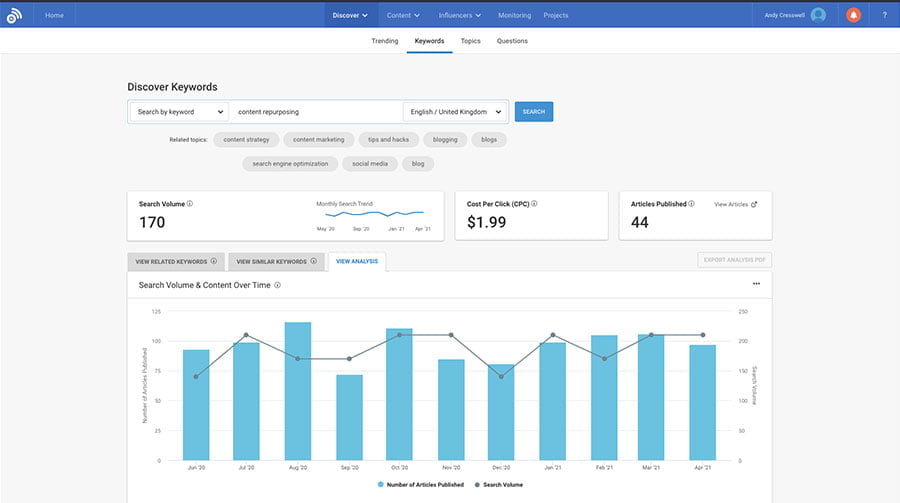This is a detailed caption for the image of a website:

The website features a sleek interface with a notable white circle adorned with curved lines radiating from it, prominently placed in the upper left-hand corner. A horizontal blue tab spans the top of the page, with white text inscribed across it. On the right-hand side, there is a generic profile image of a person accompanied by a red notification icon with white text inside. Below this, the page is sectioned into categories labeled "Trending," "Keywords," "Topics," and "Questions."

Within the "Keywords" section, which is highlighted by a blue bar, a gray subsection urges users to "Discover Keywords" and provides options to "Select by Search by Keyword," request context, repurpose content, and choose the language, with English being the default. A blue search bar is also present here, accompanied by a plethora of keywords beneath it. The search results are comprehensive, showcasing details such as a search volume of 170, a cost-per-click of $189, and 44 articles published.

A large bar graph dominates the lower part of the section, featuring bars in blue that represent various data metrics. Additionally, a black line zigzags up and down across the graph, with circles marking significant data points. This line visually represents the fluctuation in metrics, most likely denoting variations in search volume and the number of articles published over time.